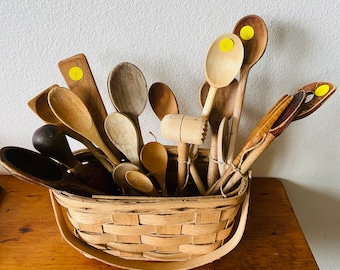This indoor photograph showcases a wooden table, brown in color, situated at the bottom of the image. Atop the table sits a light brown wicker basket shaped like a handbag, filled with an assortment of wooden kitchen utensils. The utensils include various sizes of spoons, spatulas, and a mallet, all in different shades ranging from light brown and dark brown to gray and cream. Some utensils have a black tone, likely due to their age, contributing to the color diversity. The backdrop is a clean, white wall, which provides a stark contrast to the earthy tones of the basket and utensils. This setup emphasizes the natural aesthetic of the wooden items and their assorted designs and sizes.